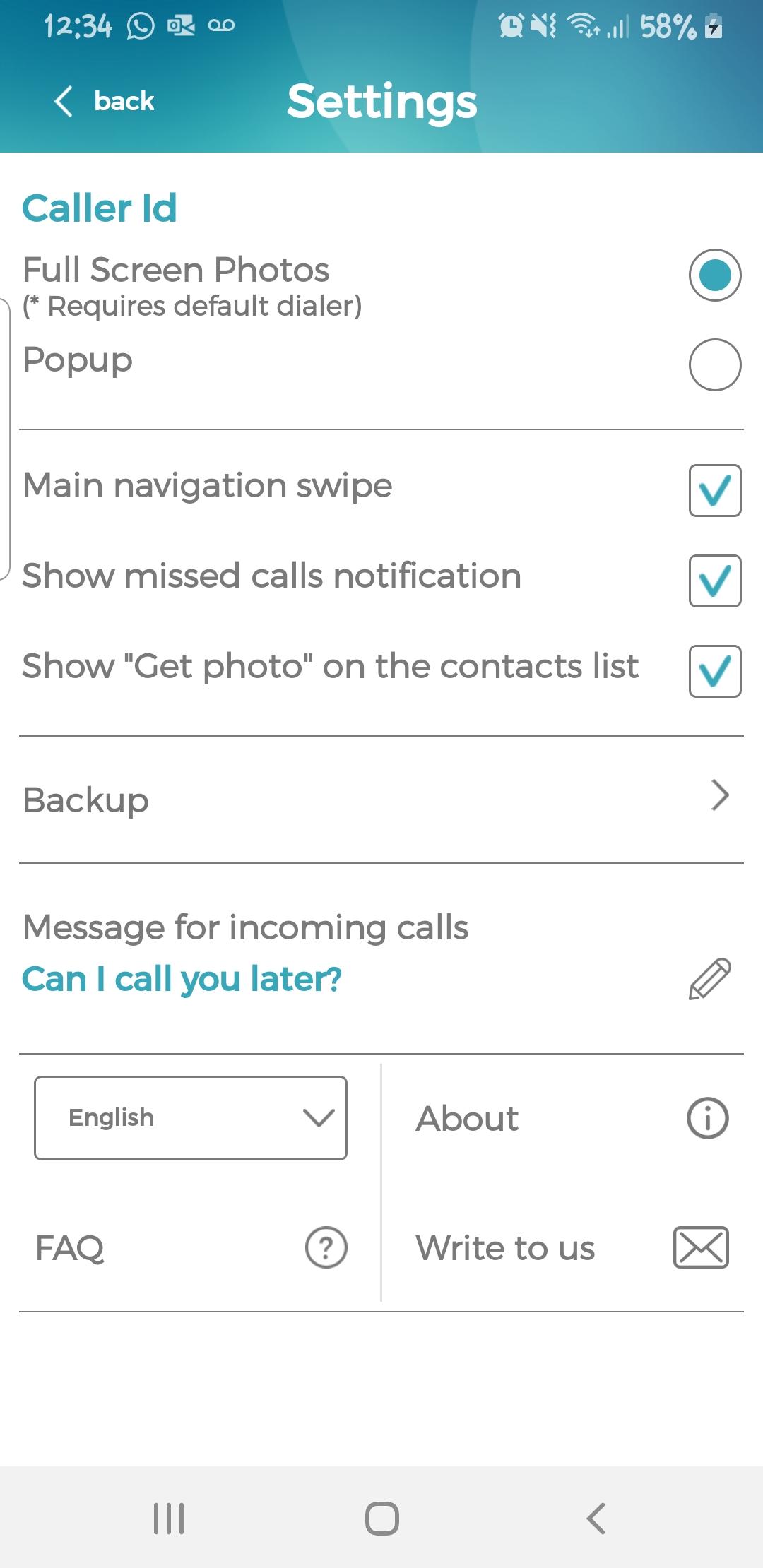The image depicts the settings screen of a smartphone, showcasing various options within the "Caller ID" settings. The battery level is indicated at 58%, with a strong network connection shown. The time displayed on the phone is 12:34 PM. A green bar at the top features a back arrow on the left.

The settings area is titled "Caller ID", and beneath it are options such as "Full screen photos," which is enabled as indicated by a teal colored circle. A notation under this option reads "Requires default dialer." There is a white, transparent pop-up button next to these settings, possibly for additional options or actions.

A bracket groups several options together: "Main navigation swipe," "Show missed calls notifications," and "Show contact photos in the list," each of which is checked, indicating they are activated. Further down, there is a "Backup" section with an arrow pointing to the right, suggesting that more options are available within it.

Another section features a customizable message for incoming calls, currently set to "Can I call you later?" and this option is highlighted in blue with a pencil icon indicating it can be edited. Language preferences are shown with English selected and the option to choose from a dropdown menu. Additional options at the bottom include "FAQ," "About," and "Write to us," represented with an envelope icon, likely for contacting support or providing feedback.